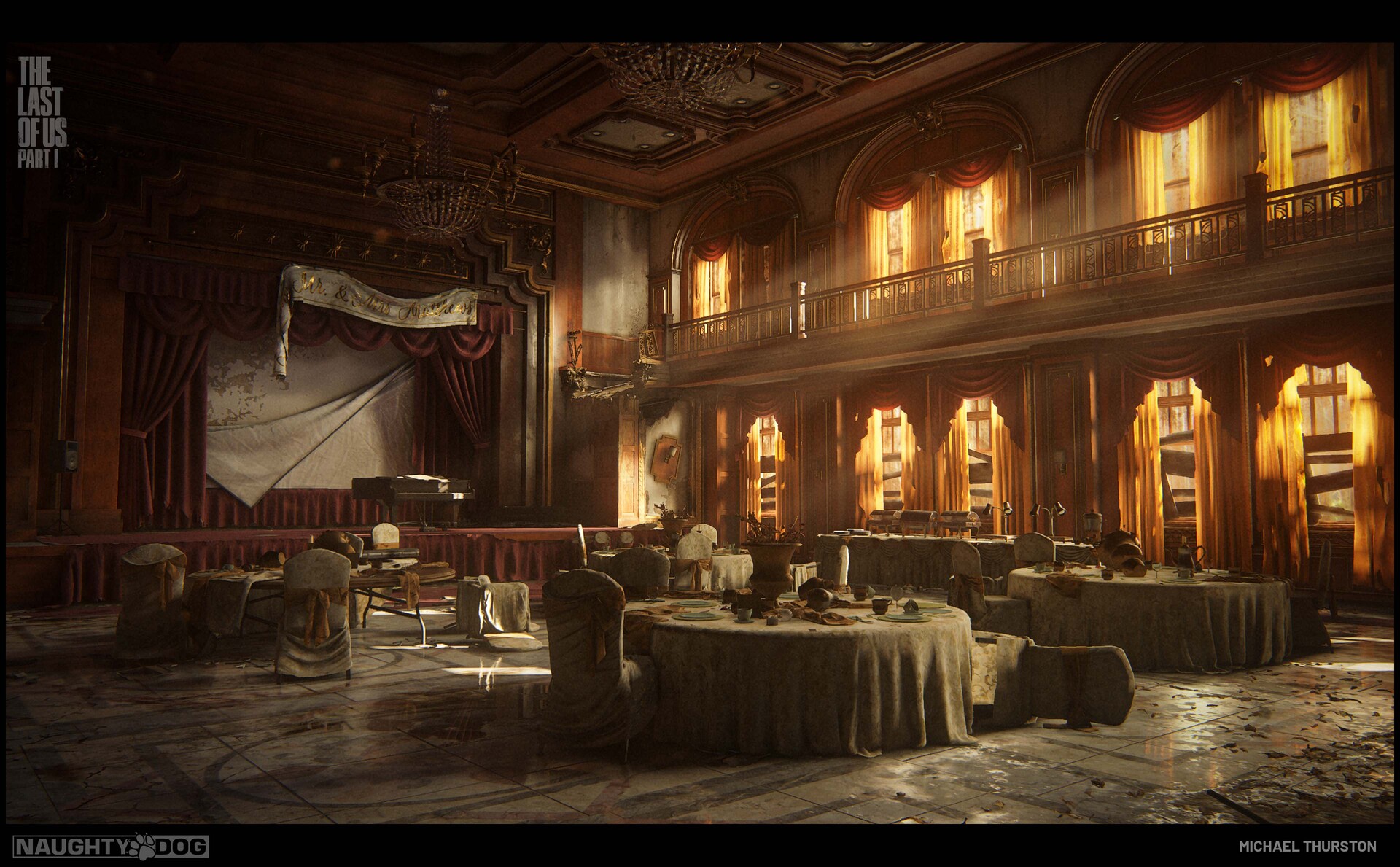This image depicts a dilapidated indoor theater or banquet hall, which appears to be a screenshot from the video game "The Last of Us Part One," as indicated by the text in the top left corner. In the bottom left corner, the game's developer, Naughty Dog, is denoted with a paw print between the words "Naughty" and "Dog." The name "Michael Thurston" is written in the bottom right corner, potentially identifying the image's creator or a developer.

The setting is in disarray with chairs that have been knocked over, tables draped with tablecloths, some of which are overturned, and remnants of food scattered about. There's a stage on the left side where a red curtain is partially falling apart. At the top of the ceiling, a fancy chandelier with multiple lights adds a touch of former grandeur to the scene. The right side features two stories of windows and balconies, the windows looking partially boarded up, suggesting a history of abandonment and neglect. The once majestic ceiling has detailed, ornate designs, reminiscent of grand venues like the Sistine Chapel or the Fox Theater in Detroit, though it's now filthy and decaying. This eerie atmosphere, coupled with the chaos of the furniture, evokes a sense of abrupt departure and underlying catastrophe.